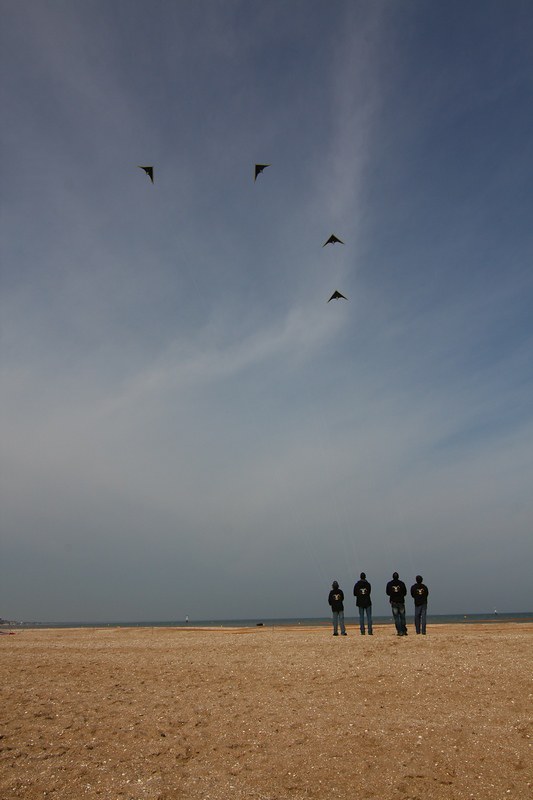The photograph features a tall, vertically-oriented composition, approximately two to two and a half times taller than it is wide. The bottom quarter of the image showcases a medium brown stretch of barren sand, resembling a desert or beach. Positioned in the center-right section of this sandy area, there are four figures appearing to be men, facing away from the viewer. They are dressed uniformly in black hoodies with a white logo or letter 'T' on the back and are all wearing jeans. Their hands are in their pockets, and they are possibly wearing dark caps, creating shadows on their heads due to the light source.

Above them, the sky occupies the majority of the image. It is a dark blue, heavily streaked with wispy, white feathery clouds stretching from the middle toward the left. In this vast expanse of sky, four black, triangular kites shaped like swallows are visible, with two flying slightly above the men’s heads, one facing upward to the left, one upward to the right and the other two slightly lower in the image. The overall atmosphere of the image portrays a serene moment of group activity, with the sharp contrast between the vast sky, the barren sand, and the identical appearance of the men against the expansive background.